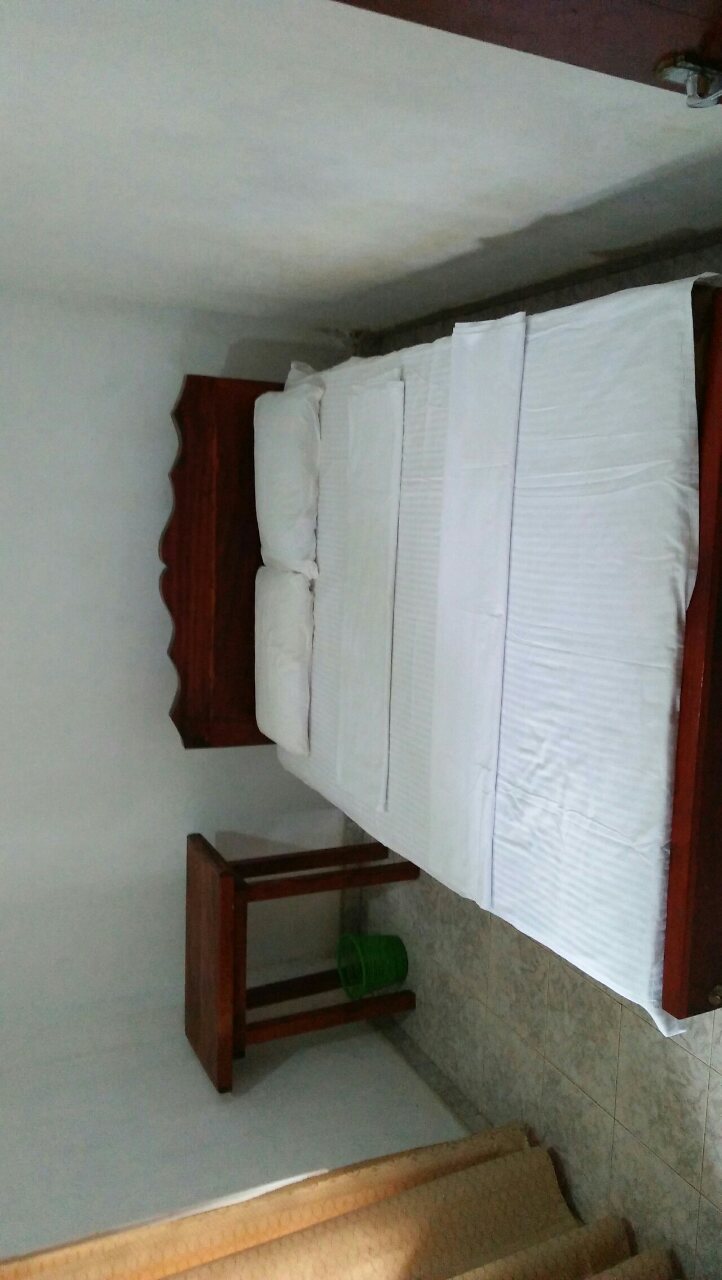This photo depicts a small, almost prison cell-like bedroom with stark, bare white walls. The room is dominated by a twin bed, which features a mahogany headboard and footboard. The bed is neatly made with white linens and includes two pillows with white pillowcases. Adjacent to the bed is a dark brown nightstand, under which sits a green bucket. The room also contains a window with tan, floral-patterned curtains through which a sliver of sunlight peeks. The floor is covered in floral tile with a gray baseboard lining the bottom. The scene is devoid of personal effects, giving it a bleak and unadorned appearance.